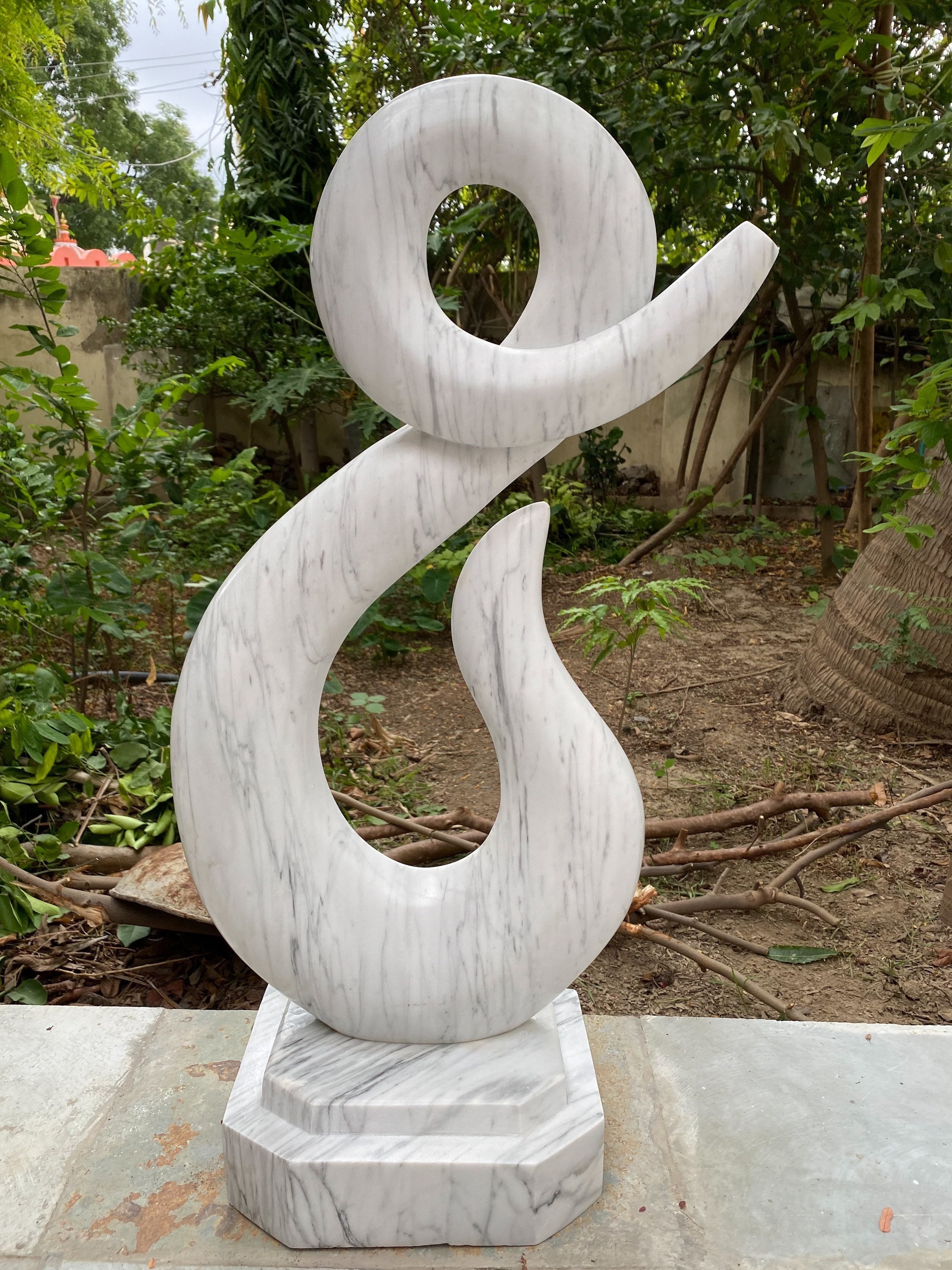The photograph features a striking marble sculpture situated outdoors, prominently displayed in a garden-like setting. The sculpture, the focal point of the image, is composed of white marble streaked with varying shades of grey, giving it a sophisticated and nuanced texture. It is intricately shaped, resembling a flowing, backward "S" or an abstract ampersand, and stands tall, capturing immediate attention. The sculpture rests on a matching squared base made from the same veined marble, which is itself placed on the edge of a cement platform. Surrounding the sculpture, the background is lush with trees, bushes, and a scatter of sticks on the ground. To the right, the trunk of a tree is visible, and in the distance, a hint of architectural structures emerges, including a roof that might belong to a pink house. The entire scene exudes a harmonious blend of natural and crafted elements, showcasing the sculpture as a centerpiece in this serene, leafy environment.